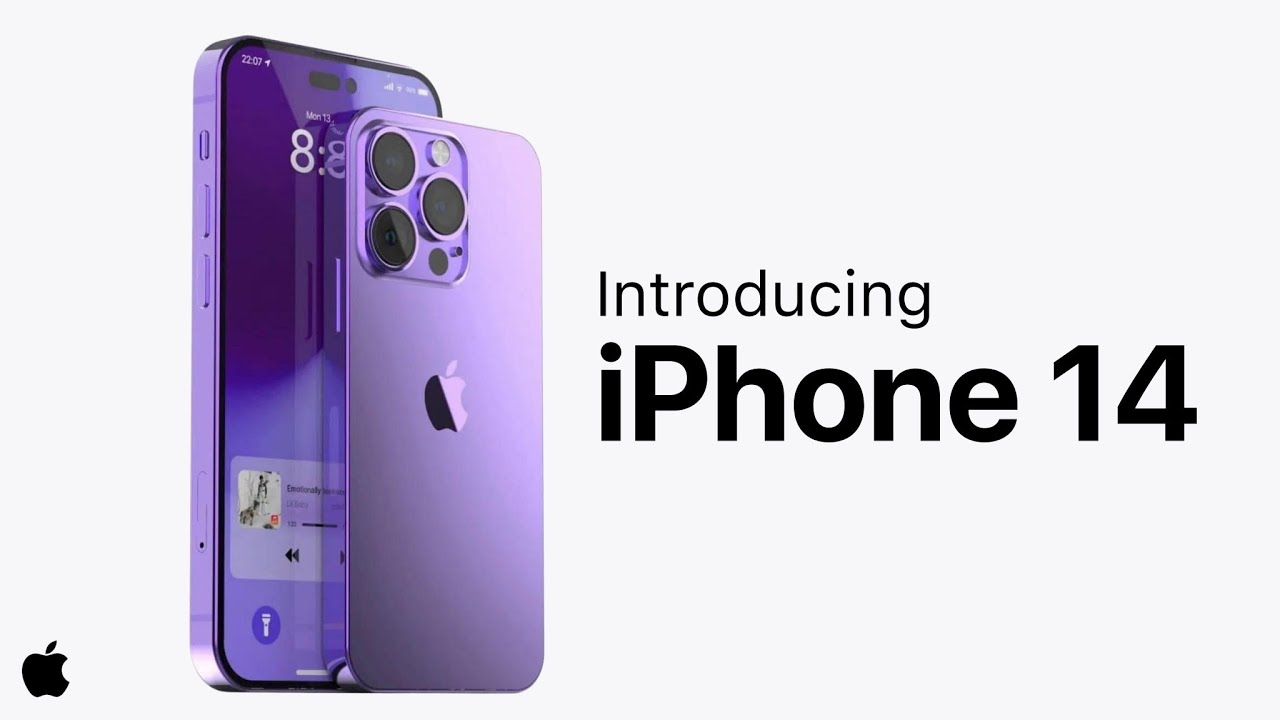Introducing iPhone 14 - A Detailed Look at Apple's Latest Innovation

This is a screenshot of an advertisement from Apple, showcasing the new iPhone 14. The background is a very light blue, almost whitish color, providing a clean and minimalist aesthetic. Positioned in the bottom left corner is the unmistakable Apple symbol, a black apple with a bite taken out of it.

The advertisement prominently features the text "Introducing iPhone 14" with "iPhone 14" displayed in larger, bolder black letters, making it stand out significantly more than the word "Introducing." To the left of this text, the purple iPhone 14 is showcased in all its glory.

The image displays the iPhone 14 from both the front and back. The back of the phone, leaning against the front, reveals its sleek design and the presence of three black camera lenses arranged neatly. The Apple symbol on the back is distinctively white and black, seemingly divided in half.

The front of the phone, although partially obscured by the image of the back, displays detailed elements of the user interface. At the top left corner, the time "22:07" is visible alongside "Monday the 13th." Additional details include the number "8," reflected in the back image of the phone. At the very bottom, the music app is open with the word "Emotionally" and an accompanying icon visible, along with the flashlight icon, indicating the user interface at that moment.

This visually appealing advertisement skillfully presents the iPhone 14, emphasizing its sophisticated design and advanced features.